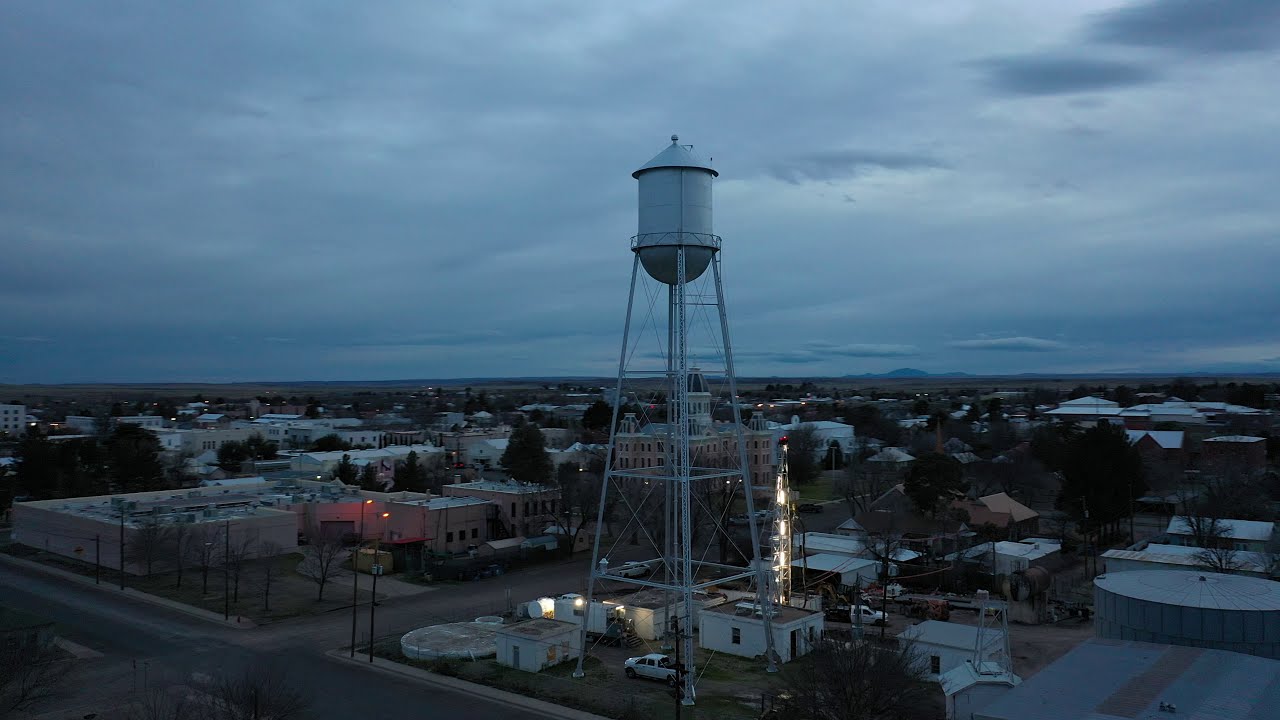This photograph captures a large, white water tower prominently positioned at the center of a small town. The town consists of low-lying buildings, primarily small warehouses, office buildings, and perhaps some businesses in an industrial area. The tallest structure, aside from the water tower, is no more than four stories high. Partially obscured behind the water tower, there appears to be a building with a domed top, possibly the City Hall. The scene is set during dusk, evidenced by the gray, overcast sky filled with black and gray clouds and the streetlights that are already on. The colors in the image are predominantly shades of blue, white, grays, and blacks, giving it a darker ambiance. No people are visible on the roads, but a truck is parked below the water tower, suggesting a maintenance area. Surrounding the central area of small buildings, the outskirts feature neighborhoods with houses. In the distant background, a lone mountain and treetops can be seen.